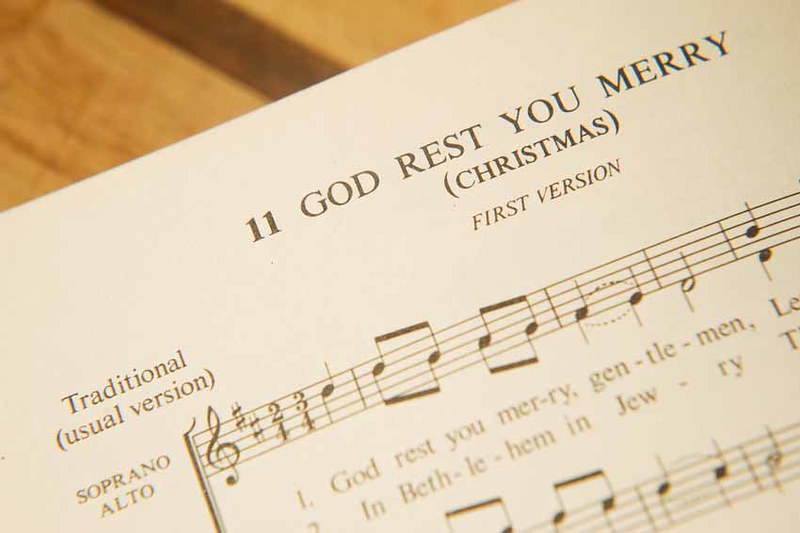This photograph captures a close-up of a piece of sheet music titled "God Rest Ye Merry Gentlemen," which is a traditional Christmas song, specifically noted as the first version. The sheet music, professionally printed in Times New Roman font, is laid on a light brown table featuring a brown stripe. The visible portion of the sheet includes musical notation, marked with treble clef symbols and time signatures of 2-4 and 3-4. The notations indicate parts for soprano and alto voices. At the top of the page, prominent text in all capital letters reads "11 GOD REST YE MERRY" followed by "(Christmas)" and "First Version" in italics. The upper left corner mentions "Traditional (Usual Version)". Only a fragment of the lyrics and notes are visible, showing partial lines such as "God rest you merry, gentlemen" and "in Bethlehem, in Jewry."